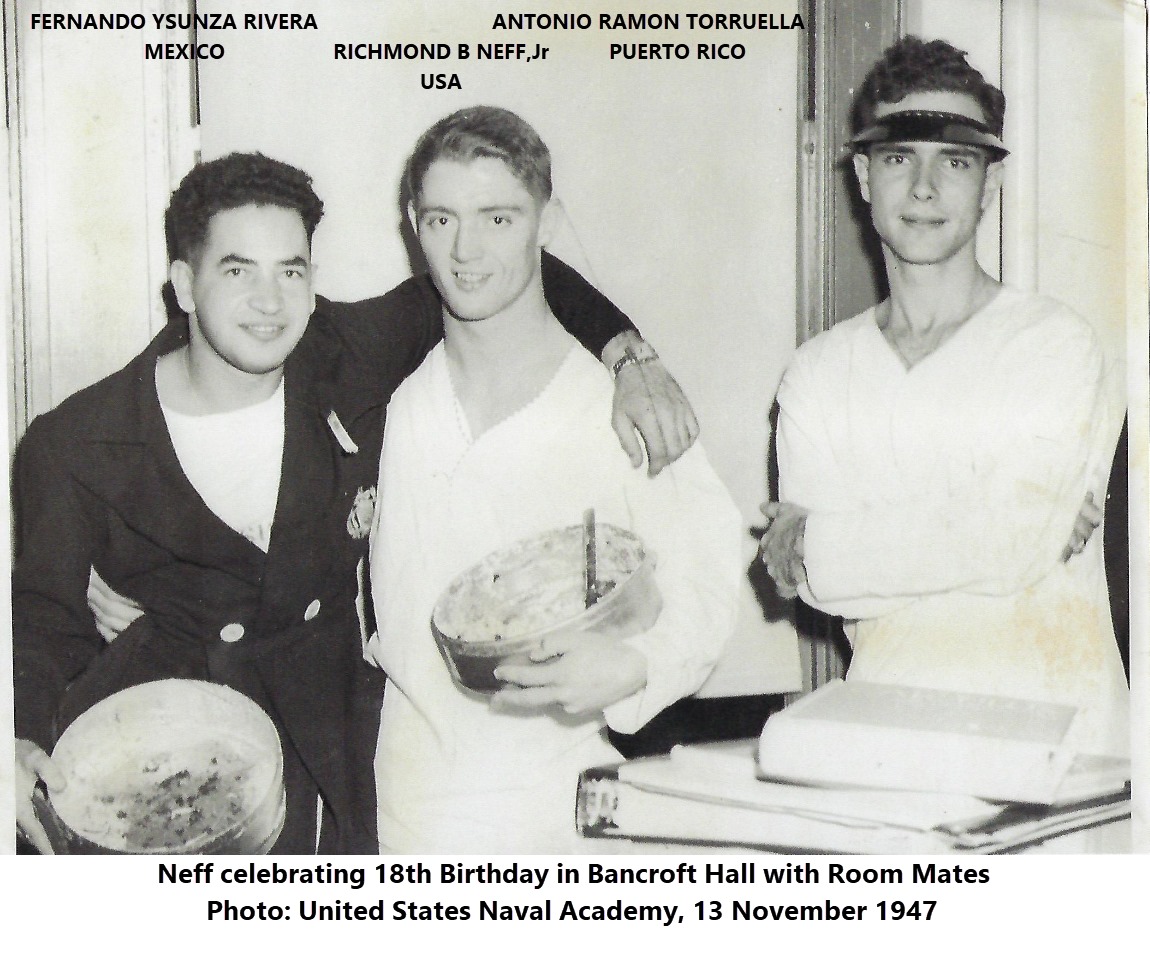This black-and-white photograph, taken on 13 November 1947 at the United States Naval Academy, captures an 18th birthday celebration in Bancroft Hall. The image features three young Caucasian men with short hair. From left to right, they are Fernando Souza Rivera from Mexico, Richmond B. Neff, Jr. from the USA, and Antonio Ramon Torrella from Puerto Rico, as labeled in the text at the top of the photo.

Fernando Souza Rivera stands on the left, smiling at the camera and holding a large round tin in his right hand. He has dark hair and is dressed in a dark blazer over a white shirt. His left arm rests on Richmond B. Neff, Jr., who stands in the center of the photo. Neff has light blonde hair and wears a white long-sleeved shirt, also holding a tin in his left hand. On the right side stands Antonio Ramon Torrella, wearing a dark visor and a white long-sleeved V-neck shirt, with a stack of books or notebooks placed in the foreground.

The caption at the bottom reads: "Neff celebrating 18th birthday in Bancroft Hall with roommates. Photo: United States Naval Academy, 13 November 1947." The photograph displays a timeless quality, showcasing the camaraderie and youthful exuberance of mid-20th-century naval cadets.